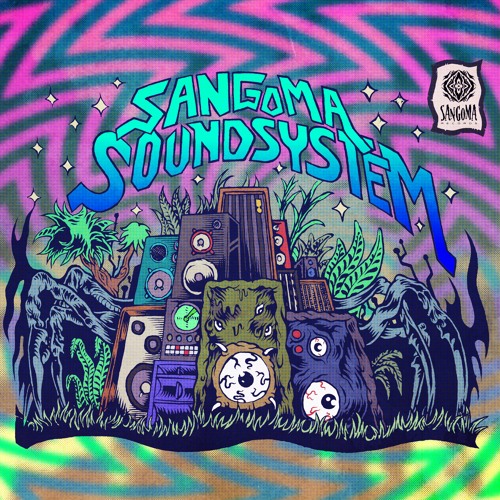The image is a vibrant, neon-colored illustration resembling a trippy band poster, possibly the front cover of a vinyl record or CD. Dominated by a psychedelic theme, the background features swirling pink lines and zigzag patterns in purple, black, green, yellow, and blue pastel shades. Central to this animated, graffiti-styled scene is the text "Sangoma Sound System," rendered in neon blue writing that fades into darker blue, with accompanying stars. The poster is populated by numerous cartoonish, neon-colored speakers, some brown, green, or blue, often featuring monstrous faces with red, veiny eyeballs where the speaker cones should be. Black figures lurk around the speaker towers, adding to the eerie vibe. Surrounding the base of this chaotic audio setup is a border of light grass under a black overlay, accentuating the trippy green and blue patterns beneath. In the top right corner, a small tag reiterates the "Sangoma Sound System" logo.